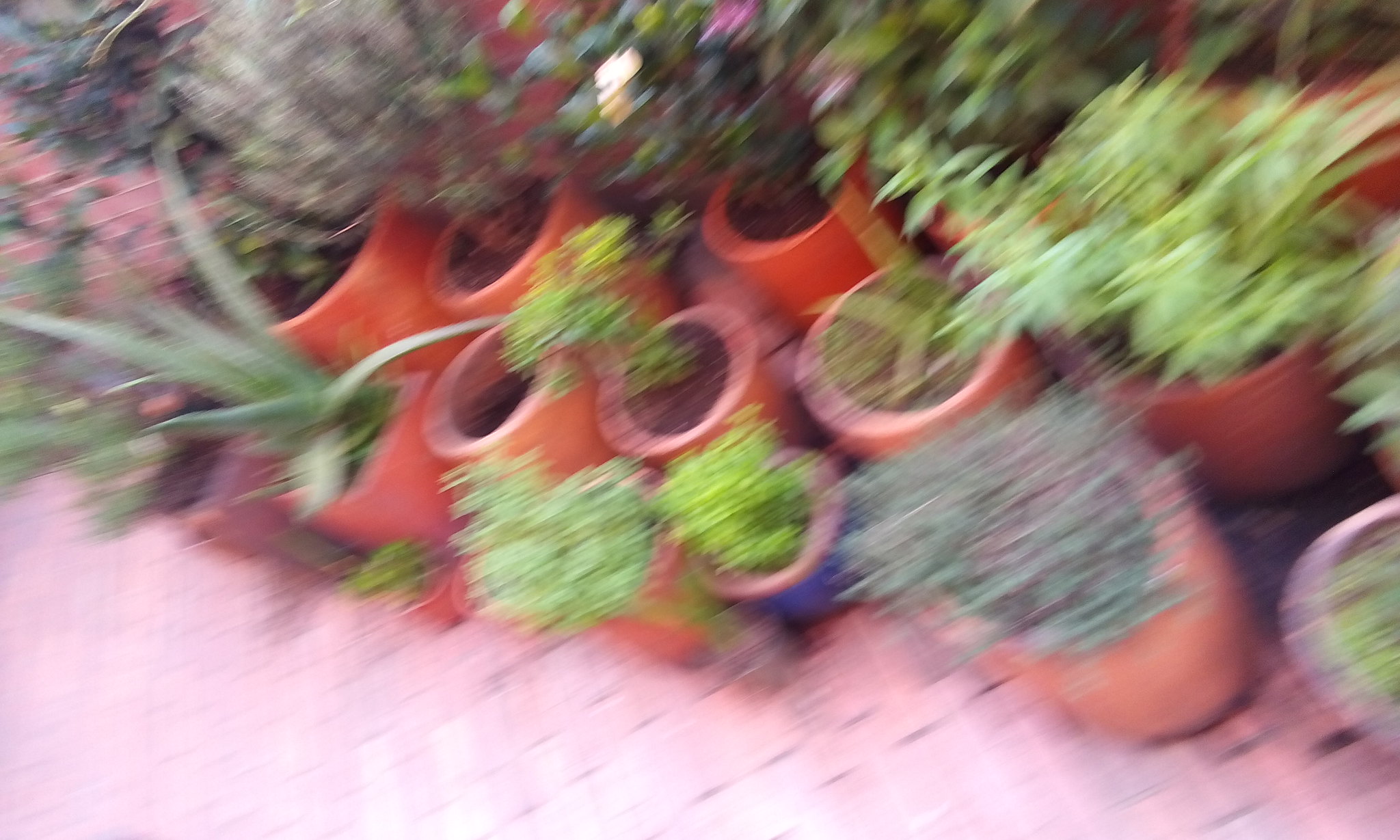The photograph captures an angled, downward view of a partially visible garden area. The image is notably blurry and out of focus, which adds a sense of mystery and organic texture to the scene. The bottom left corner of the photo, extending towards the right, features a red brick platform on which several plant pots are placed. The pots, predominantly orange terracotta, hold various small plants. One standout pot near the bottom center is a blue ceramic piece with a terracotta rim, adding a splash of color to the earthy tones.

Among the assortment of plants, a particularly tall specimen with elongated leaves rests on the left side, resembling a cactus or agave plant. The central area hosts what appear to be herbs and small shrubs, contributing to a diverse assortment of greenery. In the top left, a tree branch with dark green foliage and pink-hued leaves arches into the frame, adding a touch of delicate color. Nearby, a robust lavender plant makes its presence known.

Additionally, a red brick walkway is visible in the background on the left side, and it appears more in focus compared to the brick platform in the foreground. However, the overall image maintains its soft and blurry aesthetic, gently blending the elements into an impressionistic tapestry.